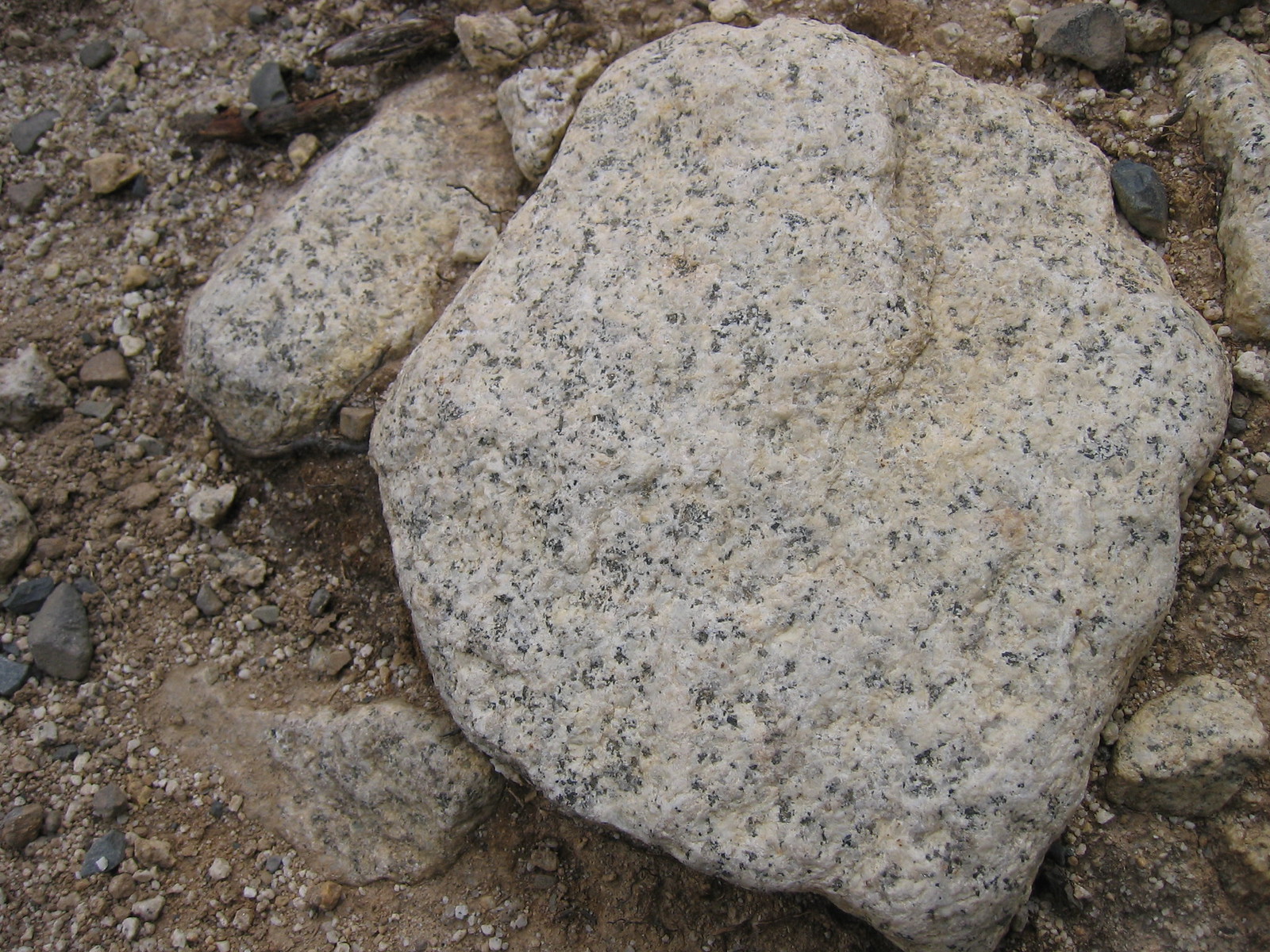The photograph, rectangular in shape, captures a shoreline scene abundant with rocks of various sizes and colors, set against a backdrop of sand and dirt. The landscape features an assortment of pebbles, medium-sized stones, and larger boulders in hues ranging from light gray, white, and dark gray to brown. Dominating the center of the image are two large, striking boulders. The larger of the two boulders is predominantly off-white, adorned with black and gray specks, and exhibits a rugged surface. This boulder is so massive that it cannot be moved by hand, and it is positioned in an upright manner on an inclined bank leading towards the water. Nearby, a smaller, oval-shaped boulder, about one-eighth the size of the larger one, shares a similar speckled pattern of black and gray and features a fine crack on its right side. The surrounding terrain, comprising darker brown soil, suggests recent moisture, contributing to an inhospitable surface for barefoot traversal, thereby highlighting the likely proximity to a hiking trail or a beach.